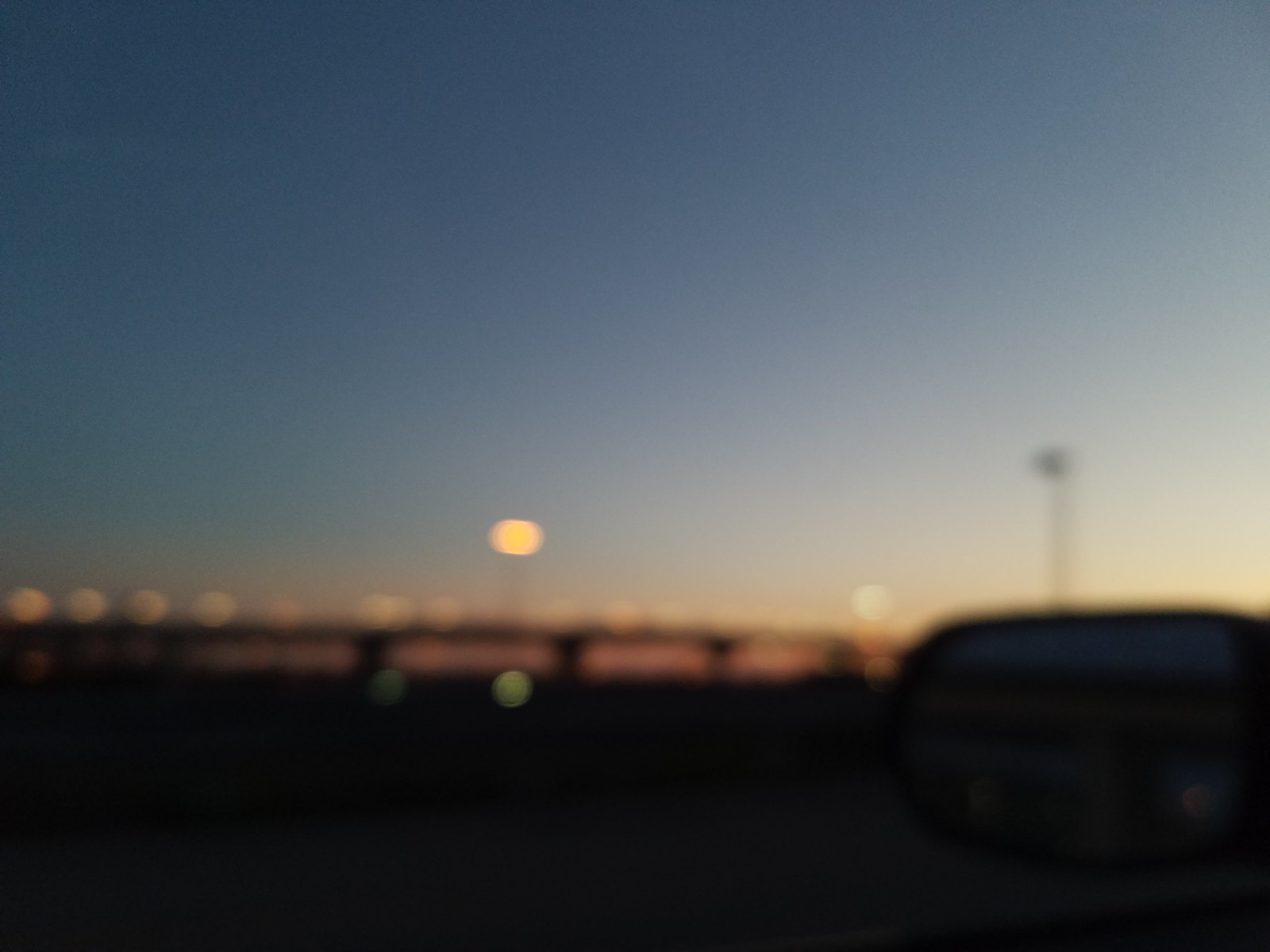This square-shaped image captures an outdoor scene, albeit in a very blurry, low-quality, and low-resolution manner. The sky, featuring a gradient from dark blue on the top left to a lighter blue and white on the top right, dominates the upper portion of the image. Beneath the sky, a long bridge spans the middle of the photograph, stretching from the left side to the right. Although the fuzziness of the image makes it difficult to discern specific details, the general layout suggests an expansive, open setting with the bridge serving as the central focal point.